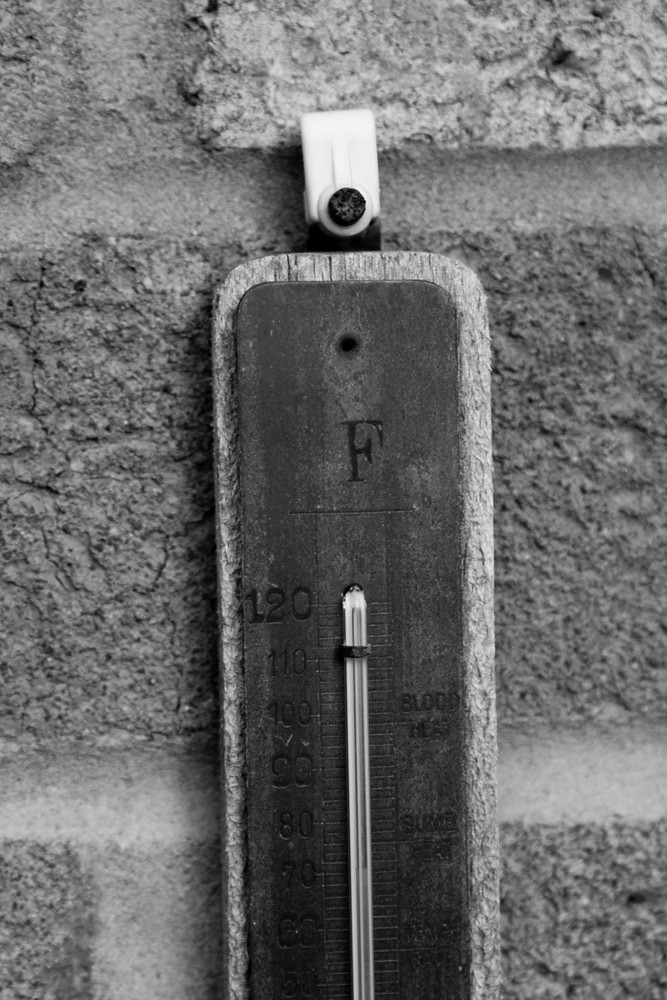A close-up of a rectangular, vertical thermometer is securely fastened to a gray brick wall. The instrument is distinctly designed to measure temperature in Fahrenheit, as indicated by the prominent capital "F" at the top. The thermometer consists of a clear, vertical glass tube, held in place by small metal hoops integrated into a flat, ruler-like structure. The dark numbering on the thermometer is clear, with the number "130" visible on its left side. Horizontal markings, likely for smaller measurements, are also present though their detail is indistinct. The thermometer is mounted to the wall using a white bracket, secured with a black screw.